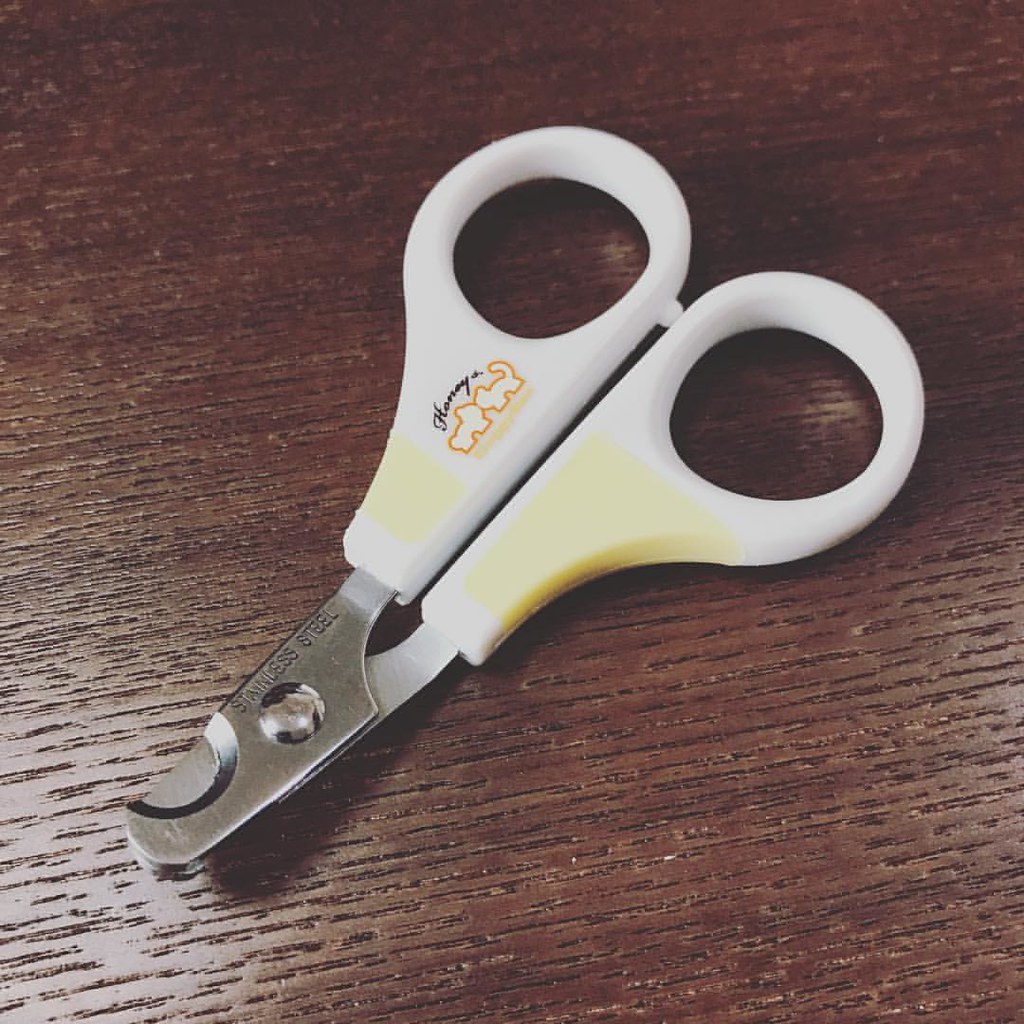This image showcases a close-up of a pair of children’s safety scissors, though they might also resemble nail clippers for pets due to their hooked blade. These scissors, around seven to eight inches long, dominate the frame. The handles are made of white plastic and feature an outline drawing of two animals, likely a cat and a dog, touching noses. Above this cute illustration is the brand name, "Honey," written in cursive. The blades are small and made of stainless steel, as indicated by the engraving near the top. The scissors are resting on a dark, engraved wooden table that adds a detailed background texture to the photo.